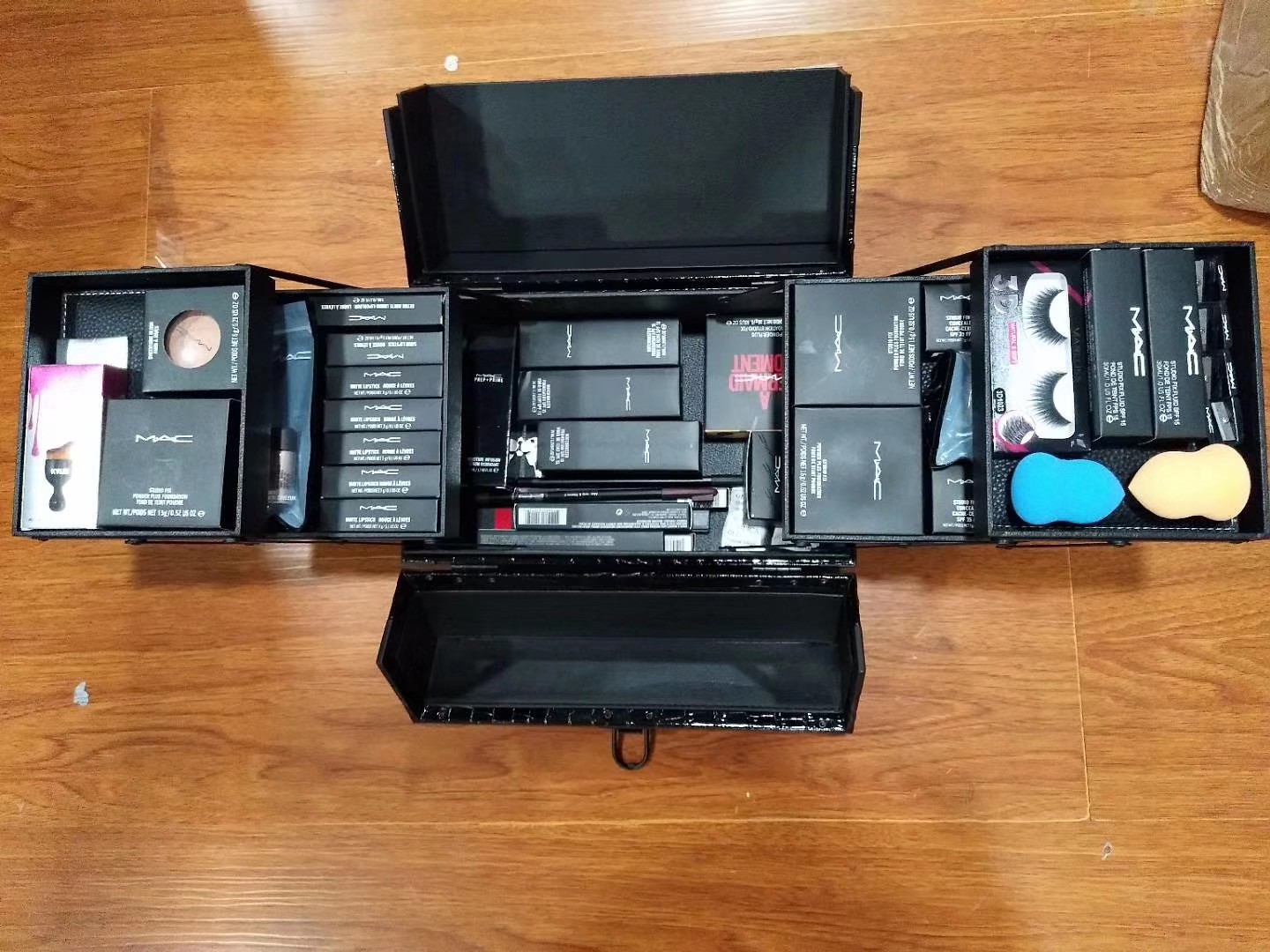The image showcases a detailed view of a makeup artist's kit placed on a brown wooden table. In the top right corner of the table, there's a piece of brown wrapped cardboard. The table itself seems to have a section in the middle that can be pulled up and out, possibly to create additional workspace.

The centerpiece of the image is the makeup artist's kit, which features a sophisticated design with a faux black crocodile print exterior. The kit unfolds into three sections on each side, resembling stair steps, while maintaining a central basin section for additional storage.

The top right section of the kit is organized with a variety of false eyelashes, multiple tubes of mascara, and two beauty blenders—one blue and one pale yellow—positioned to face each other. Moving towards the next section, it likely contains an assortment of eyeshadows, identifiable by their square shapes, along with potential eyeshadow applicators.

The central section offers a mixed assortment of items such as eyebrow pencils, additional tubes of mascara, perfume, cheek powder, and possibly other makeup essentials. The section on the upper left side appears to be dedicated to lipsticks, all neatly boxed, their colors hidden within the sealed packaging. Finally, the outermost left section contains more cheek powders and facial powders, used to cover blemishes and acne.

Overall, the kit features various MAC products, indicating either a professional affiliation with the brand or a preference for their products. Notably, all items within the kit are sealed and unused, suggesting that the makeup artist is just starting out.